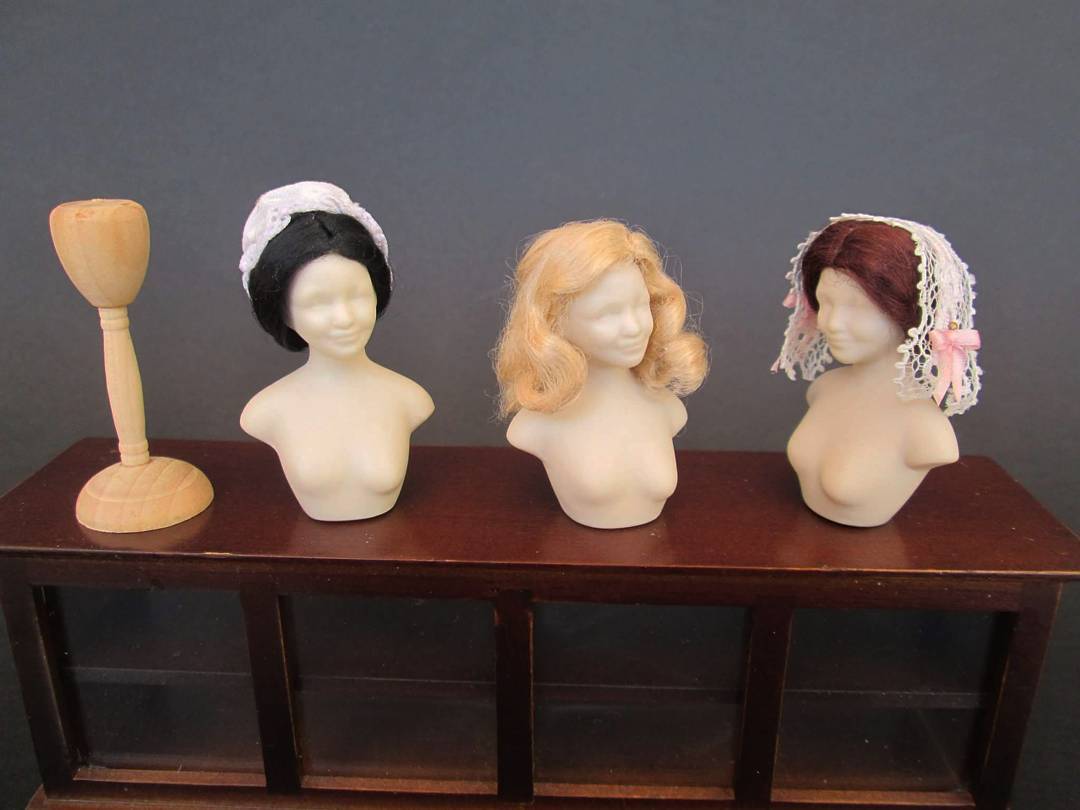In the photograph, a dark cherry wood console, possibly a hutch or an entertainment unit, is prominently displayed. The console features four glass panels with internal shelving. There are visible scrapes along the edges, revealing its worn character. Resting atop the console are three female mannequin busts, each with distinctive features. The first mannequin, positioned on the left, dons a black wig topped with a white bonnet. The middle mannequin has a long blonde wig, while the third mannequin on the right sports a red wig adorned with a crocheted, see-through lace headpiece with pink ribbons on both sides. These mannequins, showing detail from chest upward and noticeably without arms, have pale cream-colored plastic faces devoid of painted eye details. Adjacent to them, on the left, stands a wooden wig holder resembling a tall paper towel holder, but with a wider top to support wigs. The console and its inhabitants are elegantly framed by this rich, dark wood structure, exuding an air of antique charm.